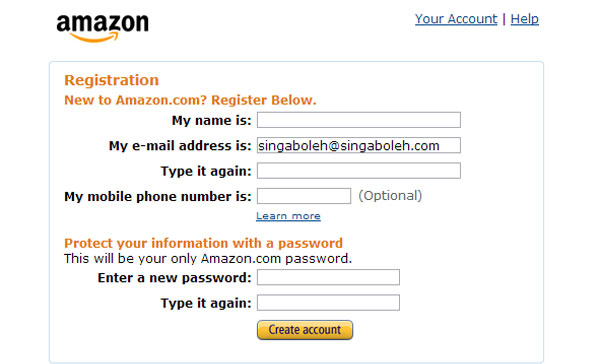The image is a screenshot of the Amazon registration page. In the upper left corner, the Amazon brand logo is prominently displayed in bold, black font with a distinct, curved orange arrow pointing to the right. On the far right corner of the image, there are clickable options in dark blue text: "Your Account" and "Help," both underlined with horizontal bars.
 
The page header reads "Registration" in orange text, followed by the subtitle "New to Amazon.com? Register below" also in orange. Below this, several fields are available for user input in bold black text: "My name is" with an accompanying text field, "My email address is" with a field and a confirmation field beneath for re-entering the email. Following this, there is a field labeled "My mobile phone number is" for users to input their phone number.

A new section titled "Protect your information with a password," written in orange, follows. It prompts users with the bold instruction "Enter a password" followed by a text field and a confirmation field labeled "Type it again." 

At the bottom, there is a gold-colored button with black text that reads "Create an account," set against a white background.